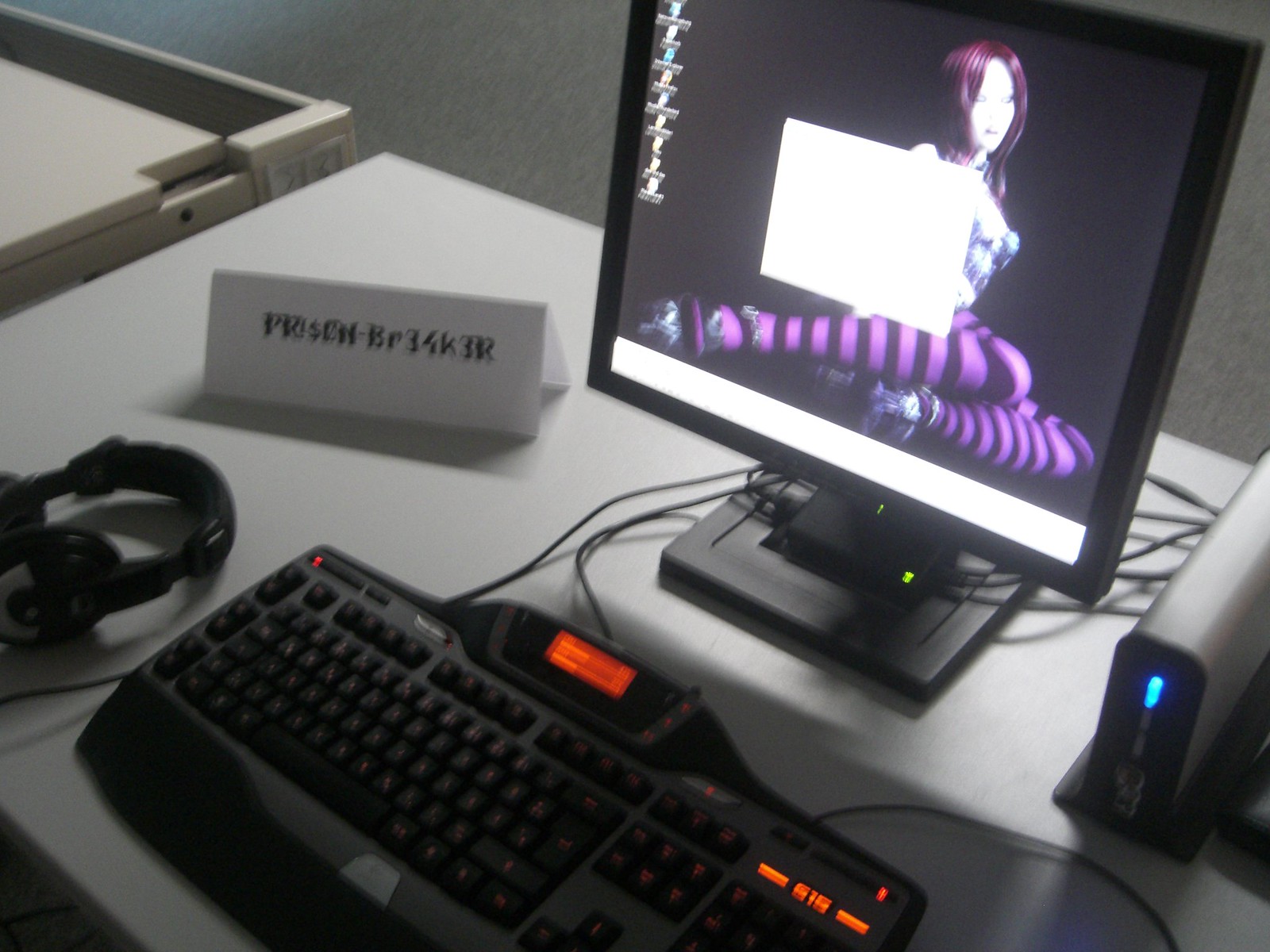This image depicts a top-down view of a modern workstation set on a white table. At the center lies a sleek black keyboard illuminated with orange lights, adding a vibrant touch to the setup. To the left of the keyboard, there is a set of headphones. In front of the keyboard sits a computer monitor displaying an animated female character with red hair, dressed in purple and black tights, sprawled against a dark backdrop. This character has some resemblance to Rihanna. Adjacent to the monitor on the right, there is a device that appears to be a router or possibly a hard drive, with numerous cables connecting it to the monitor, indicating a heavily wired workstation. Additionally, there's a small paper sign on the desk, though its text is somewhat obscured and seems to spell out something akin to “presh-br34k3r,” reminiscent of the word “berserker.” This detailed setup reflects a modern digital workspace with an emphasis on technology and entertainment.